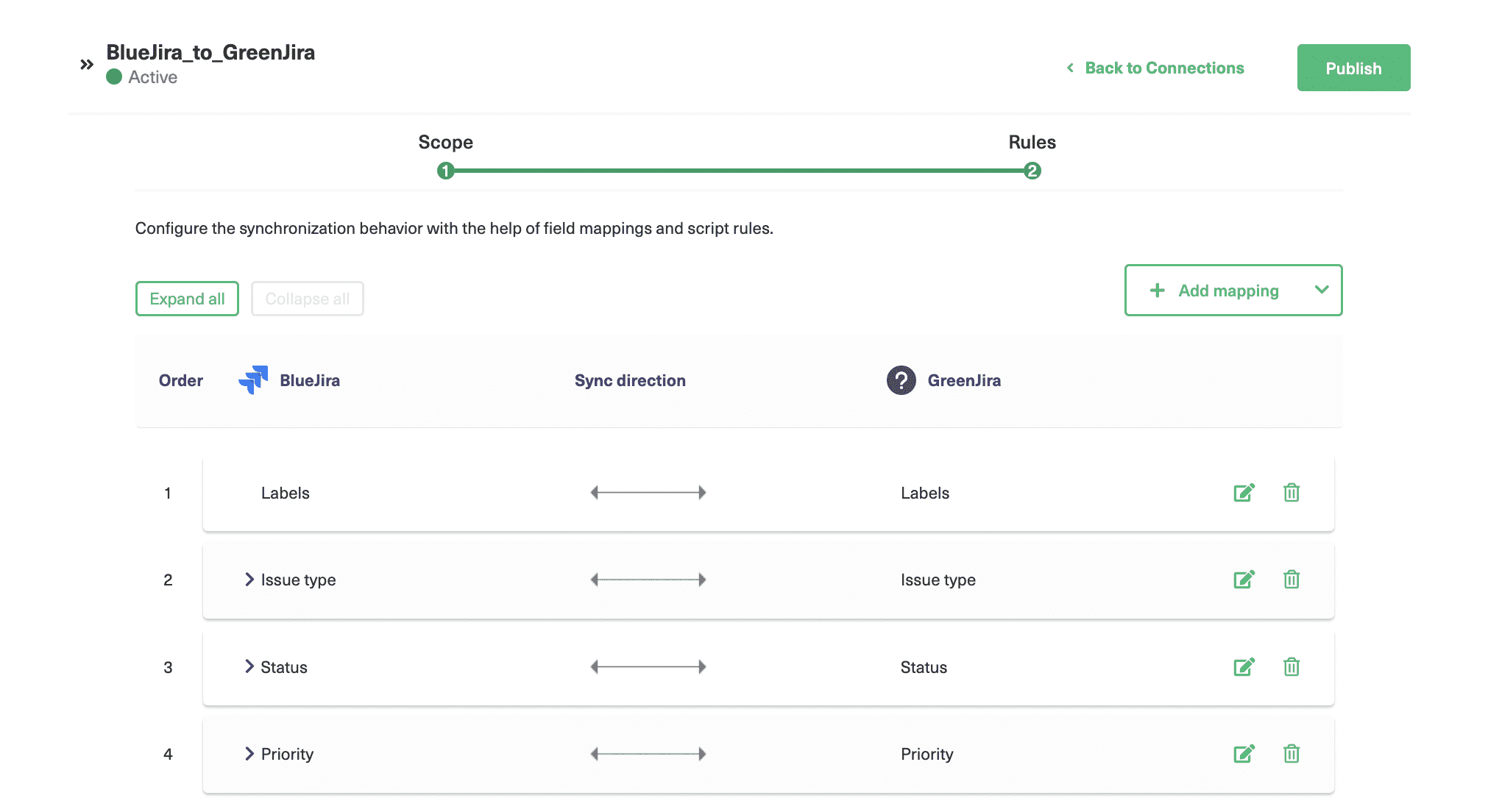This image depicts a user interface screen for configuring synchronization settings between "Blue Gyra" and "Green Gyra." The title at the top of the page reads "Blue Gyra to Green Gyra," accompanied by a green icon labeled "Active." 

Beneath this title, there is a green button labeled "Back to Connections" on the left and another green button labeled "Publish" on the right. Further down the page, the word "Scope" is displayed with the number 1 next to it, followed by a long green line that leads to the word "Rules" and the number 2.

The page includes the following instructional text in black: "Configure the synchronization behavior with the help of field mappings and script rules."

To facilitate the configuration process, there are multiple interactive buttons: a green button labeled "Expand All" and a white button labeled "Collapse All." There is also a green button with a drop-down arrow labeled "Plus Add Mapping."

The interface is divided into several sections to organize different mapping parameters:
1. **Order:** This section specifies the sequence of the mappings.
2. **Blue Gyra to Green Gyra Mapping Categories:**
   - **Labels:** Connected with arrows. Includes a green icon and a green garbage bin.
   - **Issue Type:** Displayed twice, each instance accompanied by a green icon and a green trash bin.
   - **Status:** Features a green writing icon and a green garbage bin.
   - **Priority:** Also includes a green icon and a green garbage bin.

The background of this interface is predominantly white, with black text and various buttons in green and white, providing a clear and organized layout for the user to configure synchronization settings.